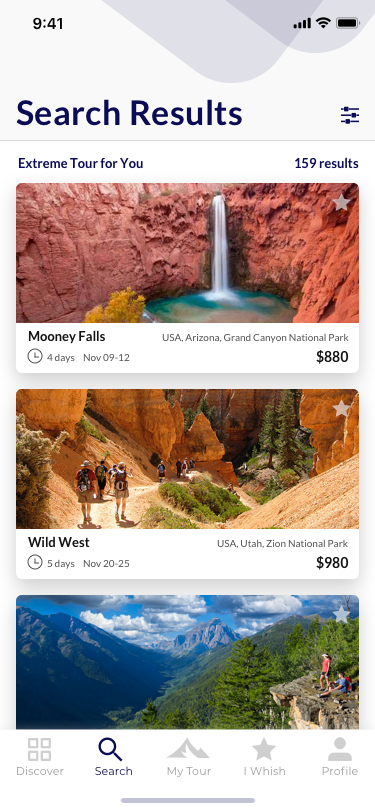This screenshot depicts a search results page for places to visit. The interface has several prominent gray-shaded areas that shape its structure. At the very top, approximately two inches of the screen are a light gray background. About an inch in from the left, a darker gray section descends two-thirds of the way down, then ascends diagonally and exits to the right. This pattern is repeated midway down the screen, creating a darker gray region where the areas overlap. In the top left corner, the time "9:41" is displayed in black, while the top right corner shows a full battery bar, Wi-Fi, and internet signals, all completely filled.

In the bottom left corner of the light gray section, the text reads "Search Results," while the bottom right corner has three horizontal sliders. Below this, a white trim about an inch thick divides the gray area, featuring the text "Extreme Torch For You" on the left and "159 Results" on the right.

The central image highlights a stunning waterfall plunging into a body of water, framed by imposing mountains. Below this captivating scenery, the left side lists the name of the place, presumably "Money Falls," with smaller text detailing its location. Underneath, it indicates the number of days stayed on the left side, and the money spent on the right.

Continuing downward, a slender gray bar separates the subsequent image. This picture captures a desert landscape with people hiking along a trail about an inch from the left edge. Mountains are visible in the distance, accompanied by sporadic bushes and trees. Directly beneath, the same format of information appears as in the previous section.

The final image shows individuals standing on a rock on the left side, overlooking a vast valley. Distant mountains and an expansive sky complete the breathtaking vista. Like before, this area provides details on the location, duration of stay, and expenses.